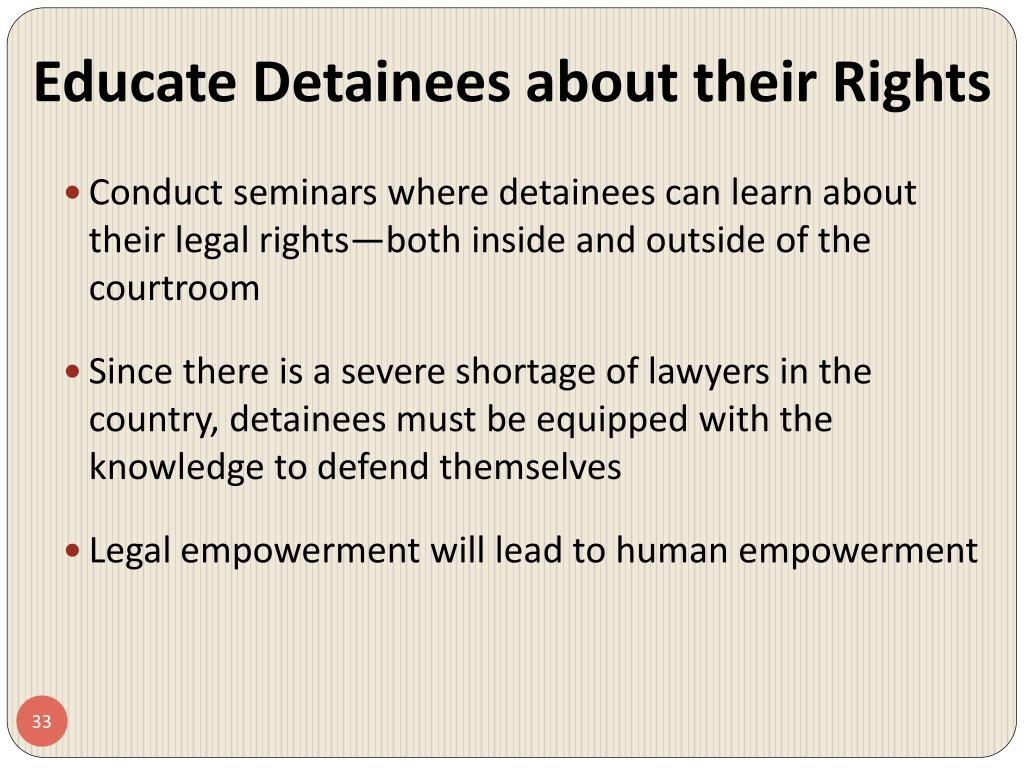The image appears to be a slide from a presentation with a lined, light grayish-tan background and thin vertical black lines. At the top, centered in black text, it reads "Educate Detainees About Their Rights." Below this title are three bullet points, each marked by a small red square and written in black text. The first bullet point states, "Conduct seminars where detainees can learn about their legal rights both inside and outside of the courtroom." The second one explains, "Since there is a severe shortage of lawyers in the country, detainees must be equipped with the knowledge to defend themselves." The final bullet point asserts, "Legal empowerment will lead to human empowerment." In the bottom left corner of the slide, there is a small red circle with the number 33 in white, possibly indicating this is the 33rd slide of the presentation.